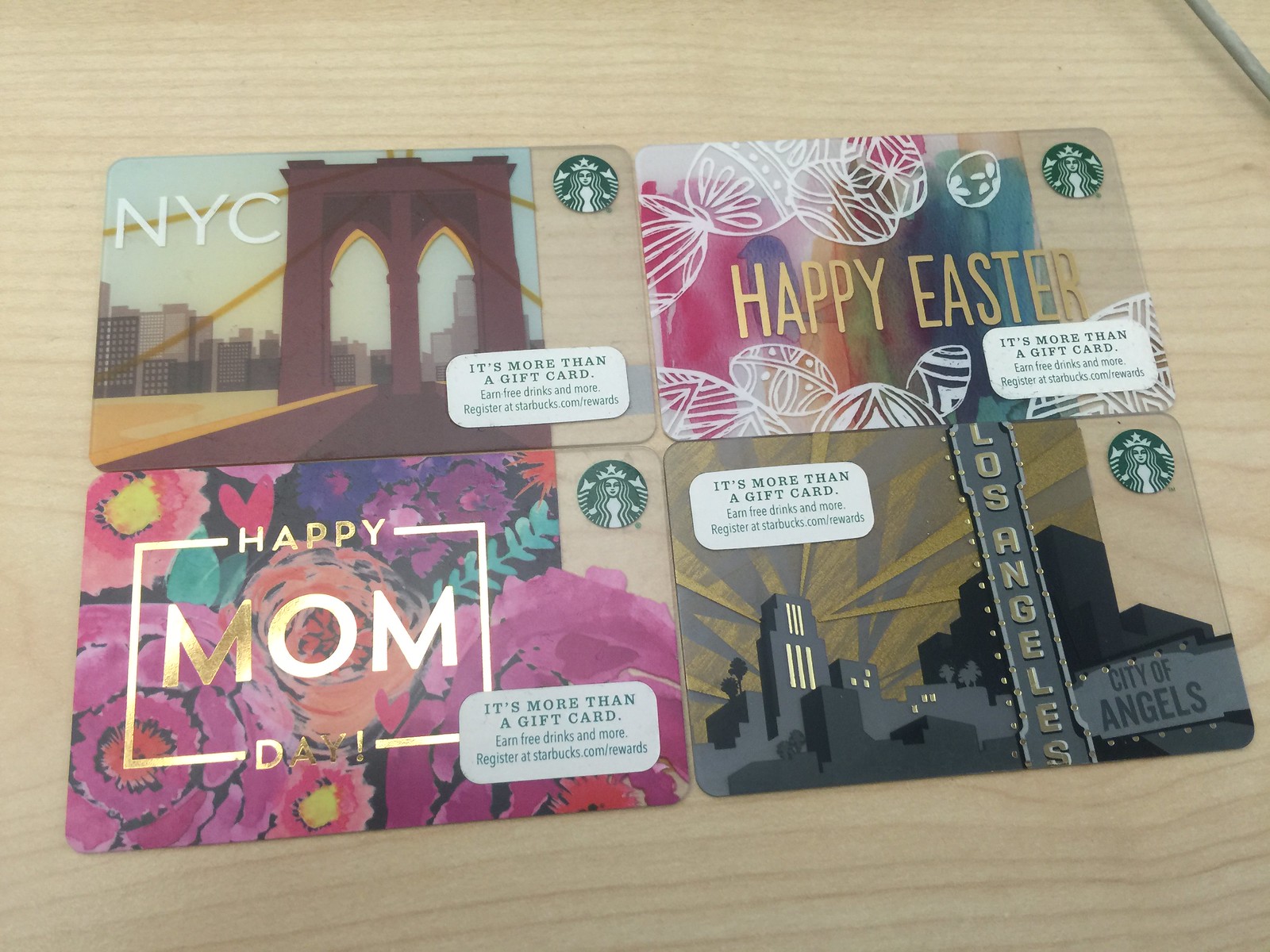The image showcases an assortment of Starbucks gift cards neatly arranged on a Starbucks counter, highlighting the variety of designs available for different occasions. Prominently featured are seasonal cards for upcoming holidays: a "Happy Easter" card adorned with vibrant pastels and elegant gold accents, and a "Happy Mother's Day" card also embellished with striking gold details against a backdrop of soft, watercolor-like paintings. Additionally, there are themed cards such as "NYC" and "Los Angeles," designed for general gifting. The "Los Angeles" card stands out with its playful use of gold tones contrasting against the sky, while the "NYC" card appears less evocative of its namesake. The overall display is colorful and eye-catching, with the gold elements adding a touch of sophistication to the festive designs.